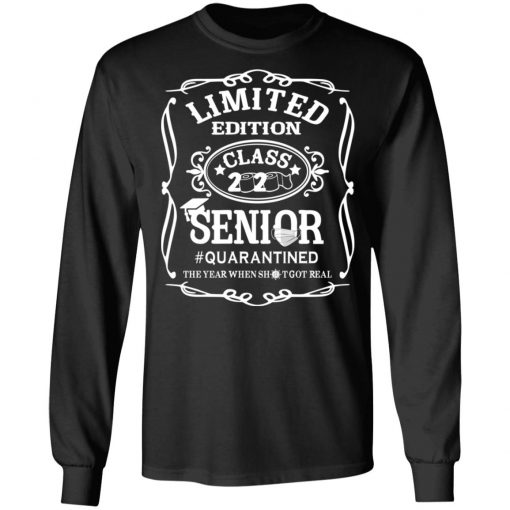The image features a long-sleeve, black T-shirt with unique and detailed graphic design. The shirt prominently displays white text and graphics in the center. At the top, it boldly reads "Limited Edition," followed by "Class of 2020" with toilet paper rolls creatively substituted for the zeros. Below this, the word "Senior" is written in large text with a graduation cap perched on the 'S'. Underneath, the phrase "#Quarantine" is featured. Following that, there is a humorous line that reads, "The year when S-H-[censored]-T got real." The entire text and graphics are enclosed in a stylized, vintage-like white border resembling a picture frame with swirly and squiggly lines. Additionally, the shirt has tighter, specially-designed wrist parts but lacks a collar. This garment humorously commemorates the unique and challenging experiences of the graduating Class of 2020.